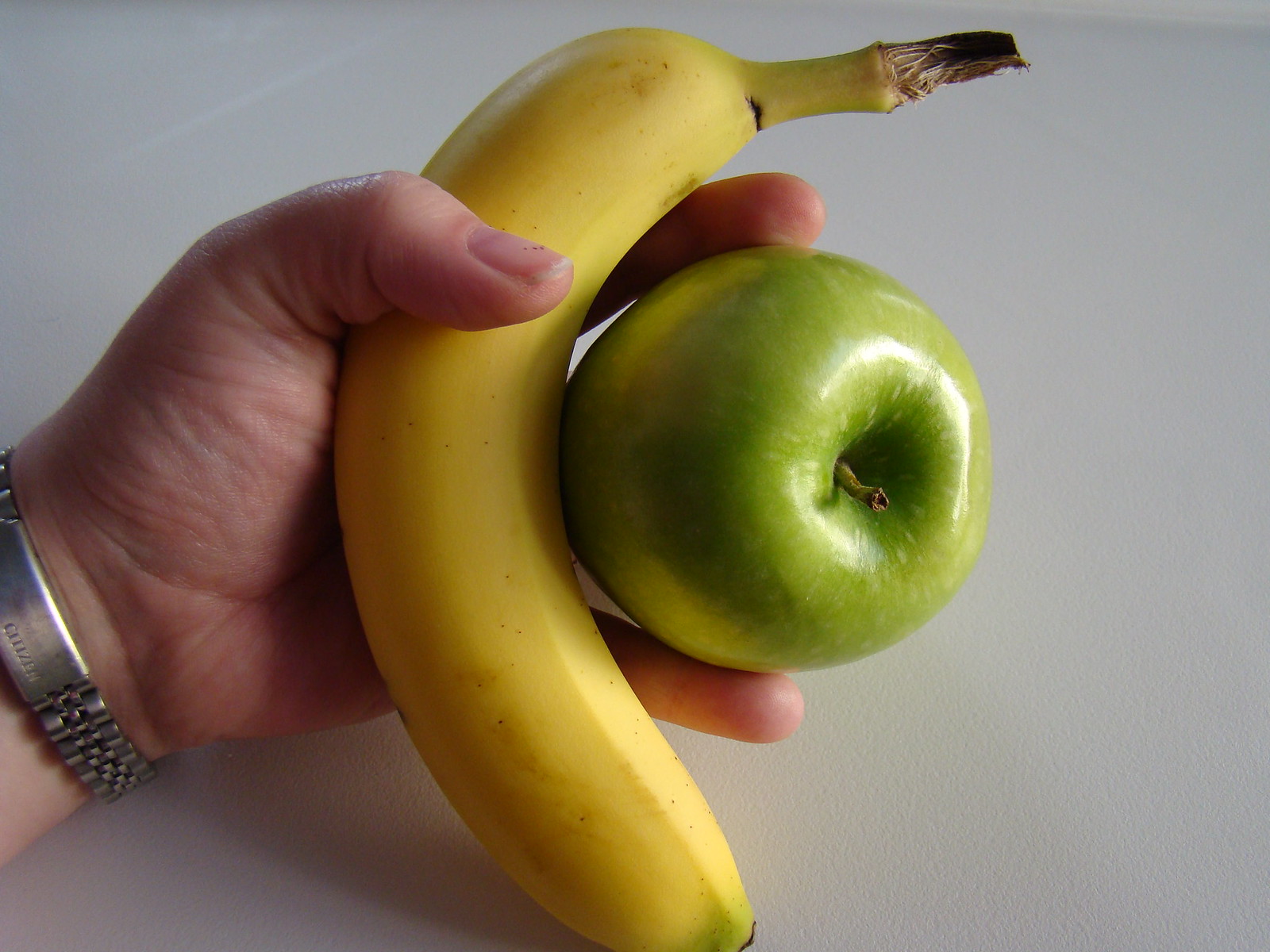In the photograph, a fair-skinned hand is prominently featured, emerging from the left side of the frame. The wrist is adorned with a watch, though only the underside is visible, revealing indistinct and blurry writing along the edge. The hand grasps a slightly bruised banana, which is predominantly yellow with a hint of green at the bottom and speckled with black spots at the top. Nestled between two fingers, a green apple is also held, with its top and stem clearly in view. The backdrop of the image is a muted gray, devoid of any text or additional elements, focusing solely on the hand and the fruits.